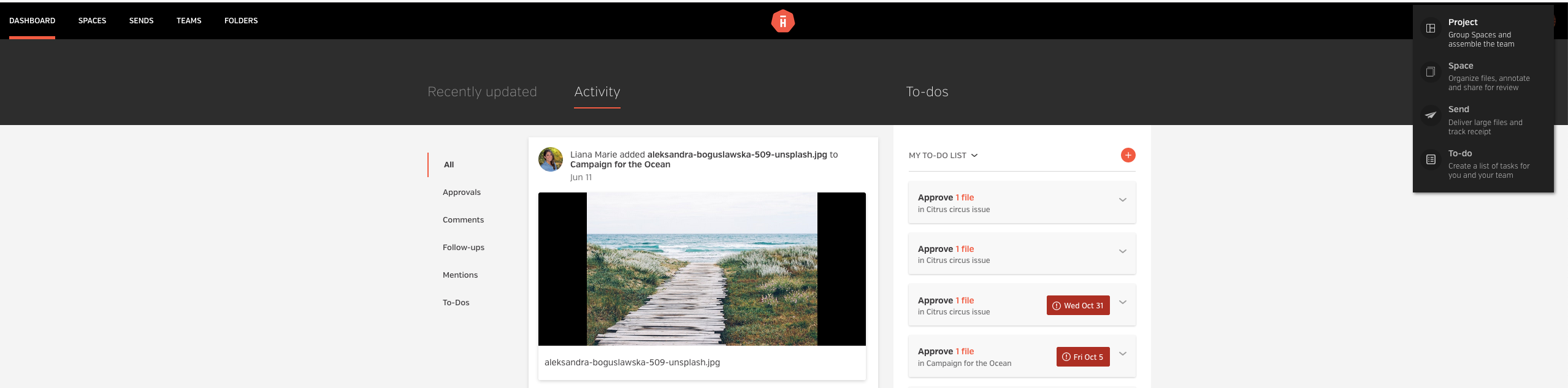The image displays a website interface featuring a top black menu bar with various navigation items, including Dashboard, Spaces, Send, Teams, and Folders. Centrally positioned on the bar is a logo: an orange hexagon encapsulating a white 'H' with a white horizontal bar across it. To the right, a drop-down menu is visible.

The main section is titled 'Project' and showcases a logo alongside the project name, "Group Spaces and Assemble the Team". Beneath this, there are several categories:
- **Space**: Organize files, annotate, and share for review.
- **Send**: Deliver large files and track receipt.
- **To-Do**: Create a list of tasks for you and your team.

Below these categories, an activity feed is present, with an update from Liana Murray who added Alexandra [unreadable] to the "Campaign for the Ocean." This feed includes a visual element displaying a boardwalk leading to the ocean.

On the right side of the image, there is a "My To-Do List" section with various listed tasks.